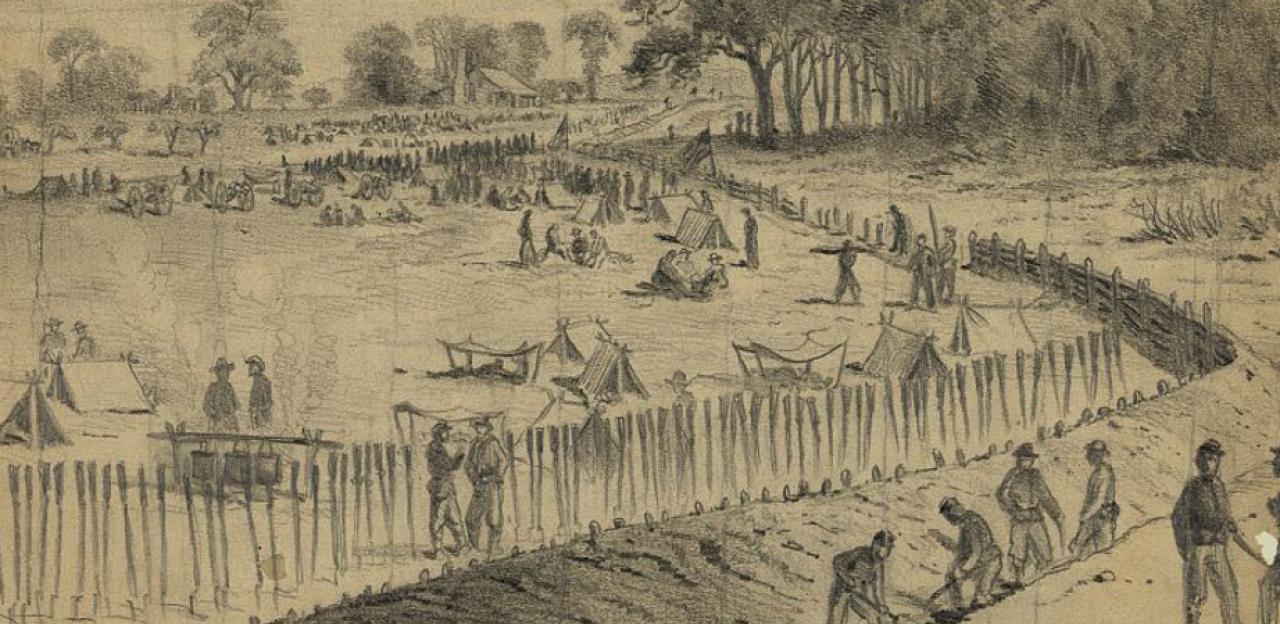The image is a detailed pencil or charcoal illustration on a faded, yellowed background, reminiscent of an old book illustration. It portrays an encampment scene, likely from the American Civil War. In the foreground, a slim-slat wooden fence runs diagonally from the bottom left, creating a perimeter around a large area filled with old-style pup tents, typical of soldiers in the 1800s. Along the bottom right, four men, possibly in uniform, appear to be digging a trench around the encampment, partially submerged in the ditch.

In the center-top area within the fenced perimeter, a crowd of soldiers is gathered, engaging in various activities such as cooking at campfires and conversing. The encampment includes scattered small cannons and a prominent American flag visible near the middle. The surrounding landscape features a tree line along the top edge, with one line of trees in the distant background separated by a field, and closer, more detailed trees occupying the right-hand side.

In the far back, amidst the field clearing, there is a house with a brick chimney, seemingly aflame. The men within the camp appear relaxed, suggesting they are setting up and fortifying the barracks rather than being in immediate battle. The overall scene exudes a sense of preparation and daily life within a wartime encampment, rendered in a monochromatic, historical style.